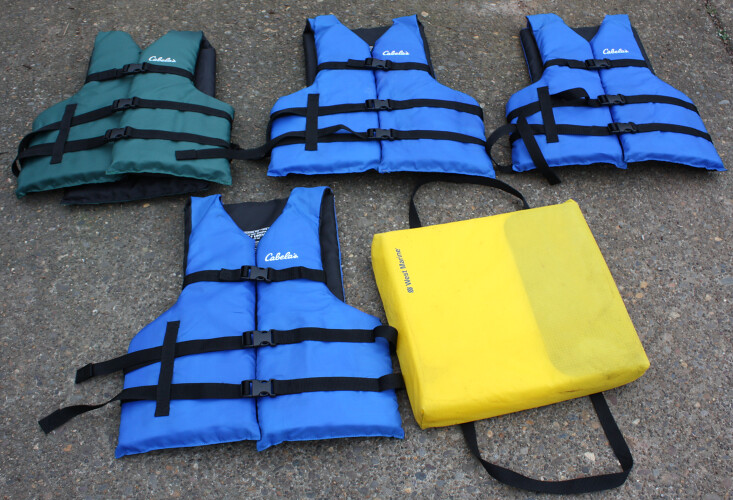The image depicts a collection of life vests and a floating seat cushion laid out on an asphalt or concrete surface. The top left life vest is a greenish-turquoise color with black strappings and dark blue or black interior, adorned with the brand name "Cabela's" in white cursive writing. Adjacent to it, on the right side, are two light blue life vests, each also featuring black straps and a similar dark interior. Below the greenish-turquoise vest is another light blue life vest with the same design elements. All life vests have identical three black straps – one at the top and two around the waist area. To the right of this bottom light blue life vest is a yellow floating seat cushion labeled "West Marine." The cushion features black looped cording around its sides and appears slightly dirty on one side.